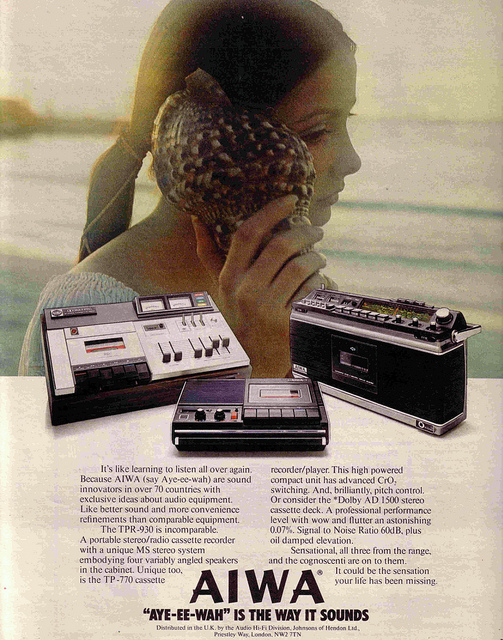The image is an advertisement featuring a mix of photography and synthesized collage elements. Dominating the top half is a photograph of a teenage girl with dark brown hair tied back in a ponytail, wearing a white shirt. She is positioned facing the right side, holding a large, speckled conch shell up to her ear, seemingly listening intently. The background hints at a beach setting, though details are blurred and indistinct. 

Straddling the border between the top photograph and the bottom section are three vintage audio devices, rendered in shades of black, gray, and brown with silver accents. These include a tape player or recorder, a stereo, and possibly a sound mixing board, each adorned with dials, tuners, and various buttons.

The bottom of the image features a stark white background. Centrally, at the very bottom, the word "AIWA" is prominently written in black text. Directly above it, in two small paragraphs of much finer black print, is additional information regarding the advertisement. The overall feel is nostalgic, blending the imagery of a youthful listener with retro audio equipment.